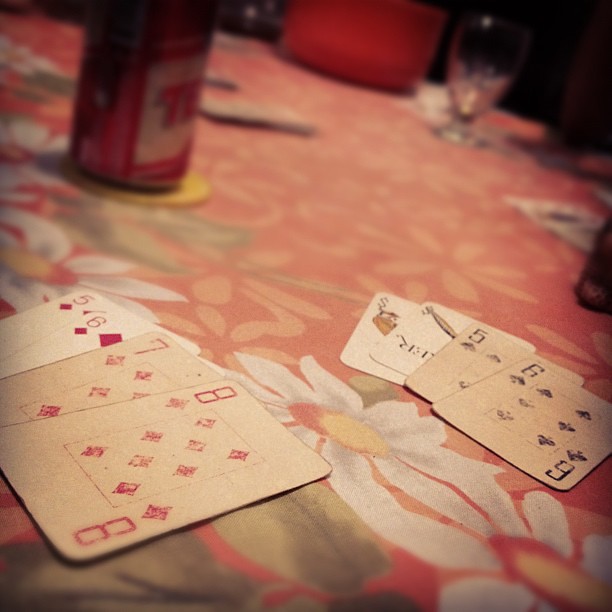This indoor photograph was taken without a flash, captured at a slight angle. At the heart of the image are two distinct sets of playing cards, positioned face up on a red tablecloth adorned with white flowers and green leaves. The first set of cards, located in the bottom left foreground, comprises the five of diamonds, six of diamonds, seven of diamonds, and eight of diamonds. Notably, the five and six of diamonds appear newer or possibly from a different deck, featuring standard modern design. In contrast, the seven and eight diamonds look aged, with a cream-colored hue and larger numbers, indicative of a more vintage design.

To the right of the image is another set of four cards. The foremost among them is a card that is difficult to identify, possibly a six of clubs due to its faded appearance. Next to it is either a five of spades or five of clubs, similarly difficult to distinguish due to its vintage look, characterized by cream-colored paper and indistinct, large numbers. Following these is a joker, only partially visible as it is upside down. The final card in this set presents an intriguing cash symbol with an unclear drawing.

Further into the background, a canned beverage, possibly soda, rests on a yellow coaster. The can is red but not distinctly branded, potentially being a Coca-Cola or Tab. Beyond this, a glass tumbler with an oval shape and narrow base is visible. The background becomes blurrier, making it challenging to discern additional details, although more playing cards might be present.